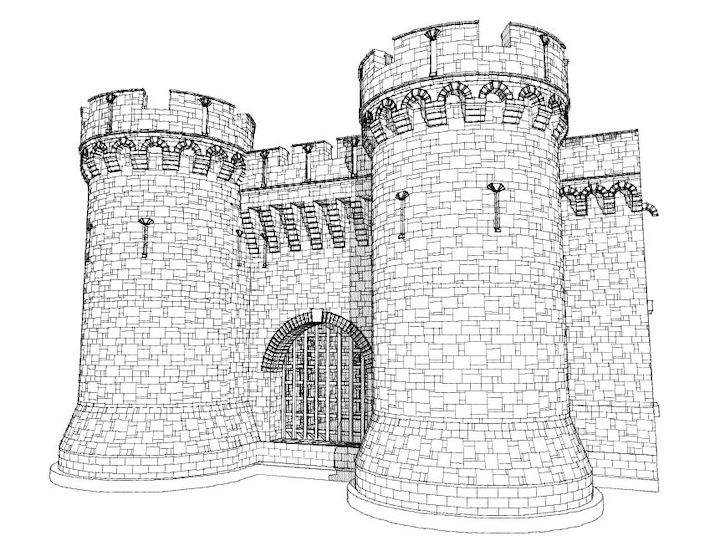The image depicts a detailed black and white line drawing of a castle-like structure. This architectural sketch showcases two prominent, turreted towers with rook-like tops, resembling chess pieces, constructed of neatly stacked rectangular stone blocks. These round columnar towers are connected by a wall, which features an arched window in the center, adorned with a heavy steel grating. The entire structure is set against a plain white background, emphasizing the intricate placement and design of each brick, contributing to the foundation of this relatively short castle building. The drawing suggests the presence of openings at the top of the towers, possibly for cannons or guns, and a large door at the base, adding to the fortress-like appearance of the scene.